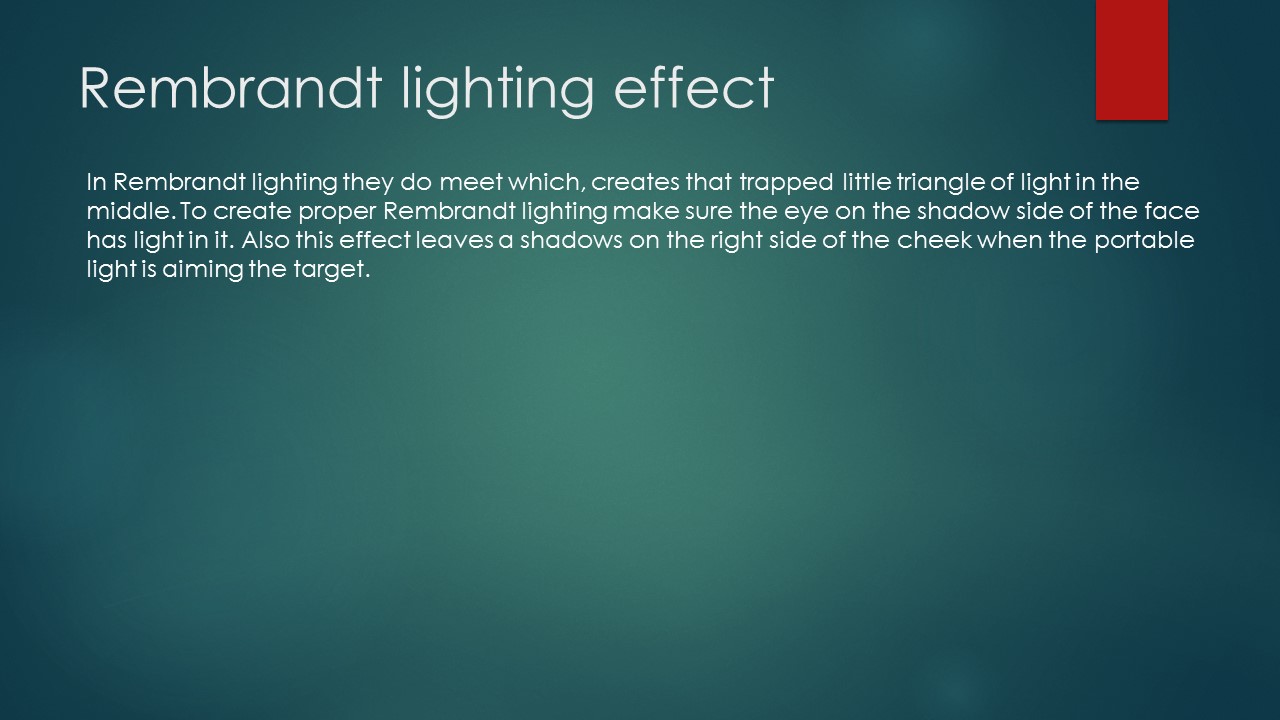The horizontal rectangular image features a striking dark green background, subtly transitioning through darker and lighter shades. Dominating the top portion is a large, bold headline in white font, declaring "Rembrandt Lighting Effect." Below this headline, smaller white text details the technique: "In Rembrandt Lighting, they do meet, which creates that trapped little triangle of light in the middle. To create proper Rembrandt Lighting, make sure the eye on the shadow side of the face has light on it. Also, this effect leaves shadows on the right side of the cheek when the portable light is aimed at the target." Adding a splash of color, a small vertical red rectangle extends about an inch from the upper right-hand corner, seamlessly aligning with the frame's edge.